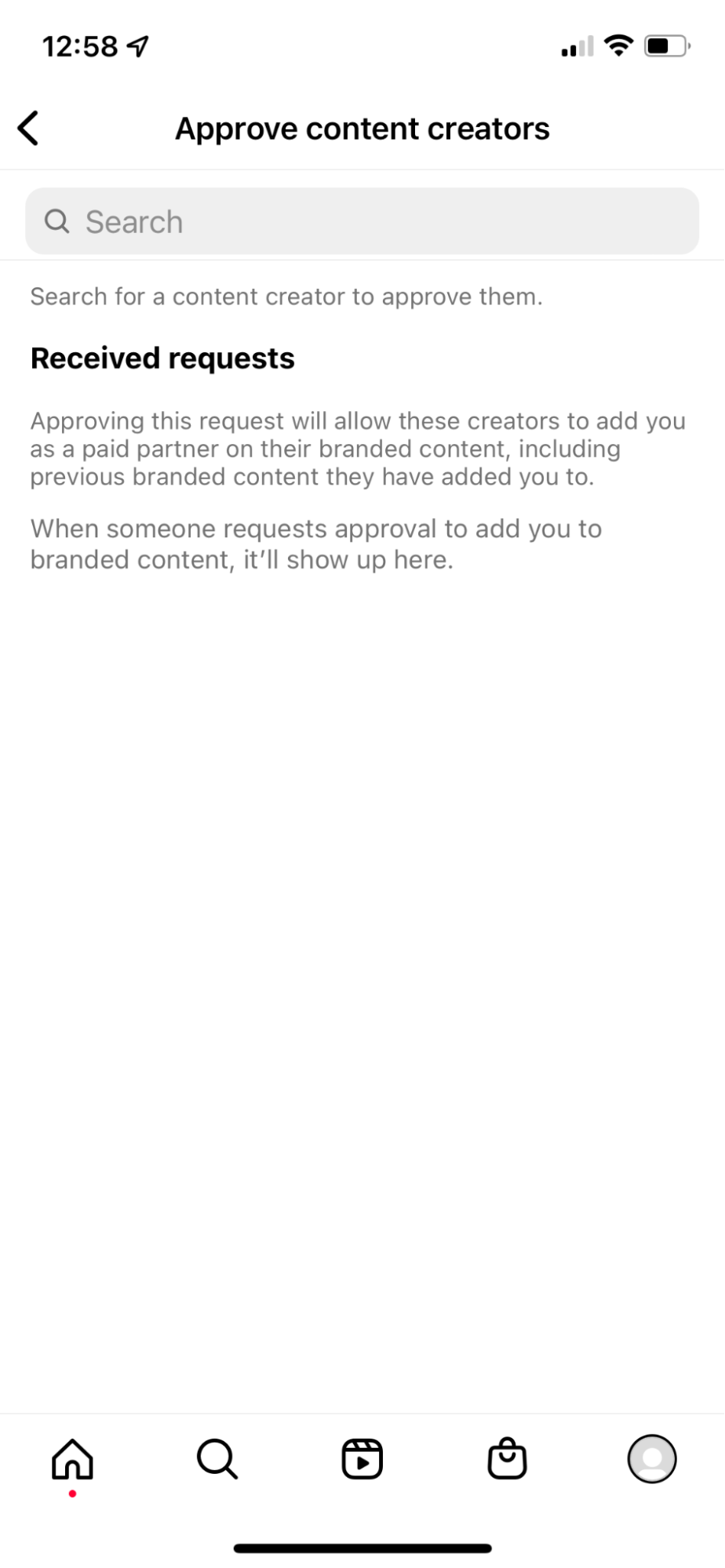A detailed screenshot of a smartphone screen shows various interface elements and search results. In the top left corner, the time is displayed, symbolic of typical smartphone layouts. To the right, a series of icons indicate the current location's signal bar strength, overall signal strength, and remaining battery life. Below this top bar, the interface indicates that a search was conducted, although the specific query is not visible. The search results display the heading "Approved Content Creators," but provide no further details on the type of content or the requesting entity. Directly beneath this, a second, seemingly redundant, search bar is present. The screen also features a section titled "Received Requests," followed by a detailed description: "Approving this request will allow creators to add you as a paid partner to their branded content, including previous branded content they have added you to. When someone requests approval to add you to branded content, it'll show up here." This context suggests the interface belongs to a platform or app designed to manage partnerships between content creators and brands.